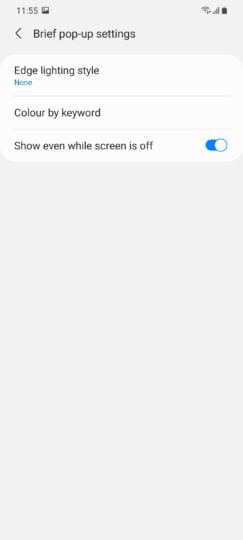Screenshot of a cell phone showcasing the pop-up settings menu. 

At the top, the time is displayed as 11:55 with an adjacent icon consisting of squares, whose function is unclear. The top right corner indicates full Wi-Fi connectivity, full network signal, and a fully charged battery. This section has a light gray background with black text.

The heading reads "Brief Pop-up Settings" with a left arrow pointing to previous settings. Below, under a similar light gray header, the screen shows a white section:

- **"Edge Lighting Style"** with black text and the current setting noted in small blue text as "None".
- **"Color by keyword"** written in black text on a white background.
- **"Show even while screen is off"** also in black text with a toggle bar beside it. The toggle is blue, indicating it is turned on.

The rest of the screen remains light gray with no additional text.